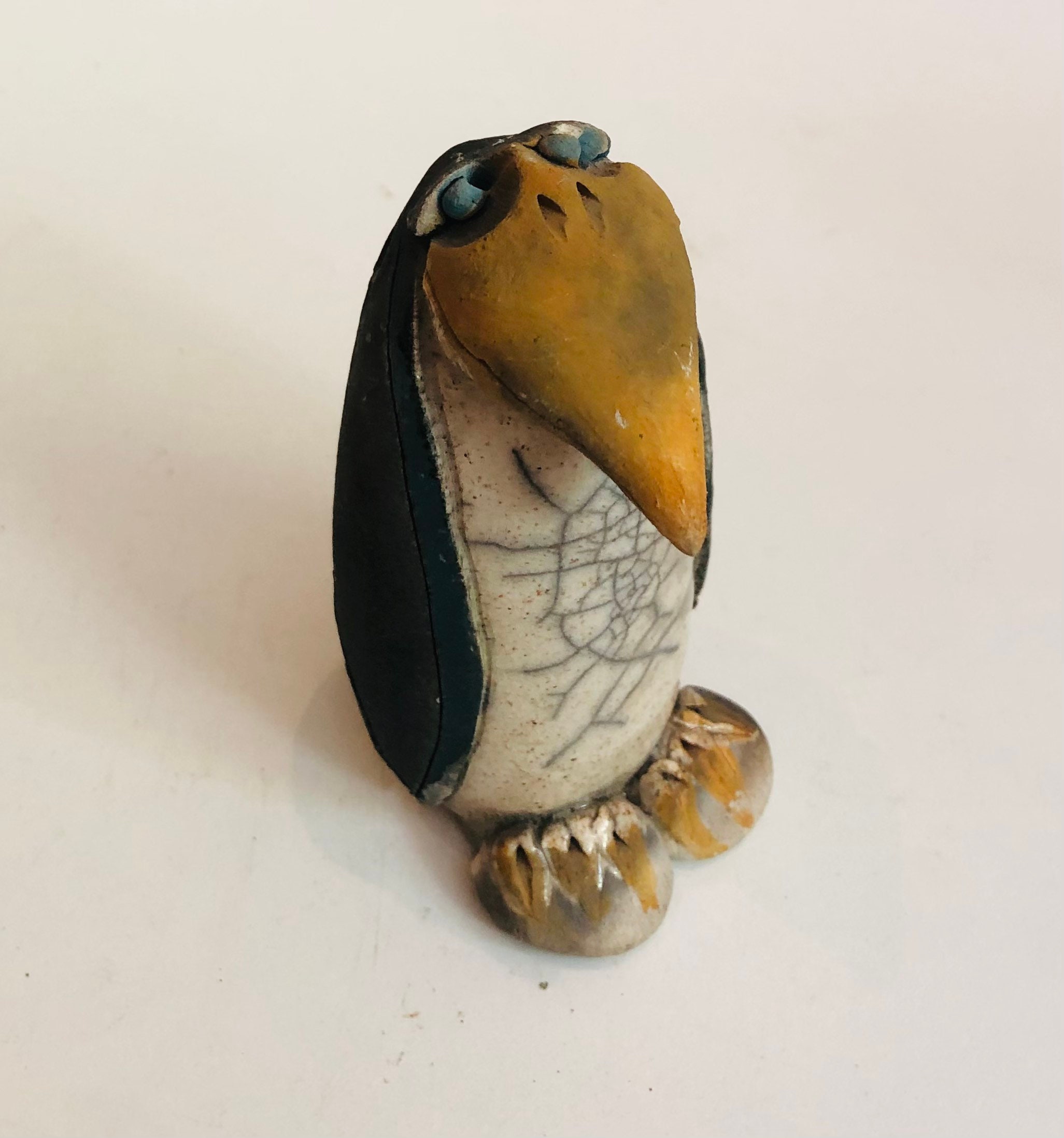The photograph showcases a charming sculpture of a penguin placed against a white background. The penguin has a white chest marked with thin lines resembling cracks or possibly drawn-on spiderweb patterns. The wings and back of the sculpture are painted black. Its feet look like circular pebbles, seemingly glued on and painted with shades of yellow and white. The penguin's beak stands out with its long, droopy form painted in a goldish or orange hue; it features nostril holes and gives the impression of having possibly been crafted from a nut. The eyes of the penguin are crafted to look like gems, grayish-blue in color, and gazing slightly upward. The sculpture has a central crack running up a significant portion of its body and casts a subtle shadow to its left, indicating some lighting in the room. Overall, this endearing penguin figure, likely sculpted from stones and creatively painted, occupies the center of the composition.